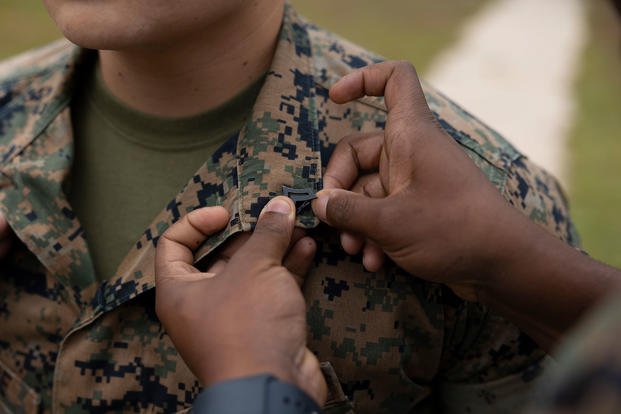The image is an up-close shot focusing on a soldier being pinned with a medal on his lapel. The soldier, whose face is not visible as the picture cuts off at his chin, has olive-colored skin with some visible freckles on his neck. He is dressed in an olive green T-shirt layered with a light tan army shirt adorned with camouflage patterns in dark green and black. The soldier stands on the left side of the photograph.

On the right side, an African American person's hands, one of which wears a black watch with a silicone band, are seen pinning a black arrow-shaped pin onto the soldier's collar. The background is slightly blurred, featuring hues of light green and white, highlighting the key moment of the medal being pinned. The main object is the soldier, centrally placed within the image, receiving the pin from the pair of hands.